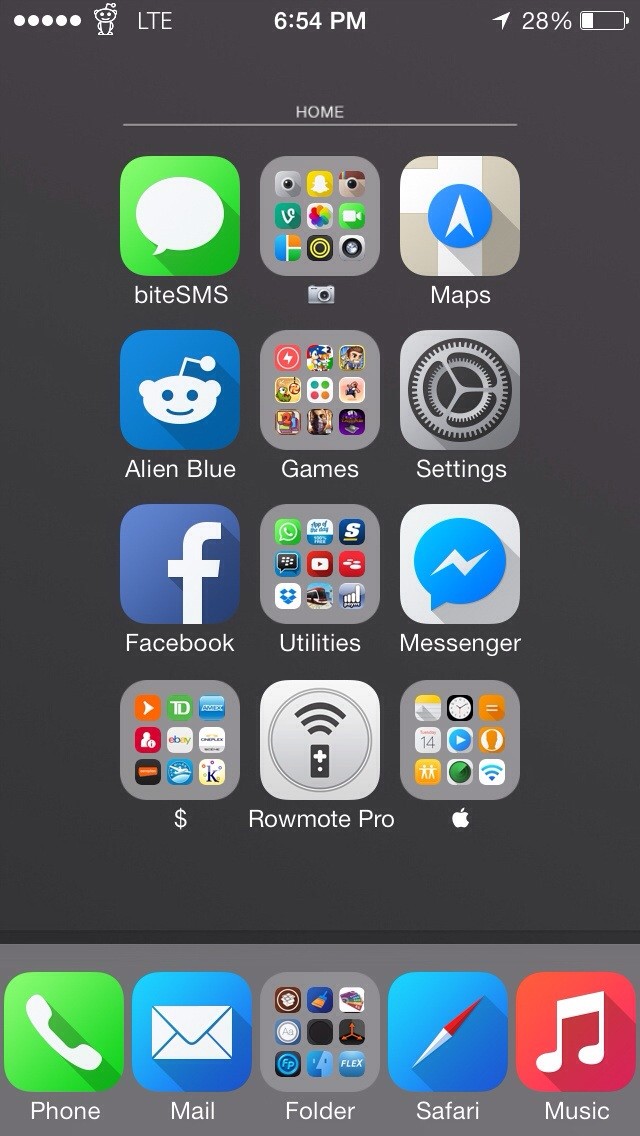This is a screenshot of an older version of an iPhone interface with a black background. At the top center of the screen, the digital clock displays "6:54 p.m." in white font. The upper right corner features a location services arrow next to a battery indicator displaying 28% remaining. To the left side, there are five horizontal white dots, indicating signal strength, next to the LTE label and a new Reddit logo.

The main part of the screen displays a grid of apps organized in a 4x3 layout, totaling four rows with three apps per row. At the bottom, there is a dock containing five apps arranged horizontally from left to right:

1. A green square icon with a white phone labeled "Phone"
2. A blue square icon with a white envelope labeled "Mail"
3. A gray square icon with multiple smaller icons grouped, labeled "Folder"
4. A blue square icon with a white and red compass arrow labeled "Safari"
5. A red square icon labeled "Music"

This detailed configuration hints at the interface design and user experience typical of earlier iPhone versions.